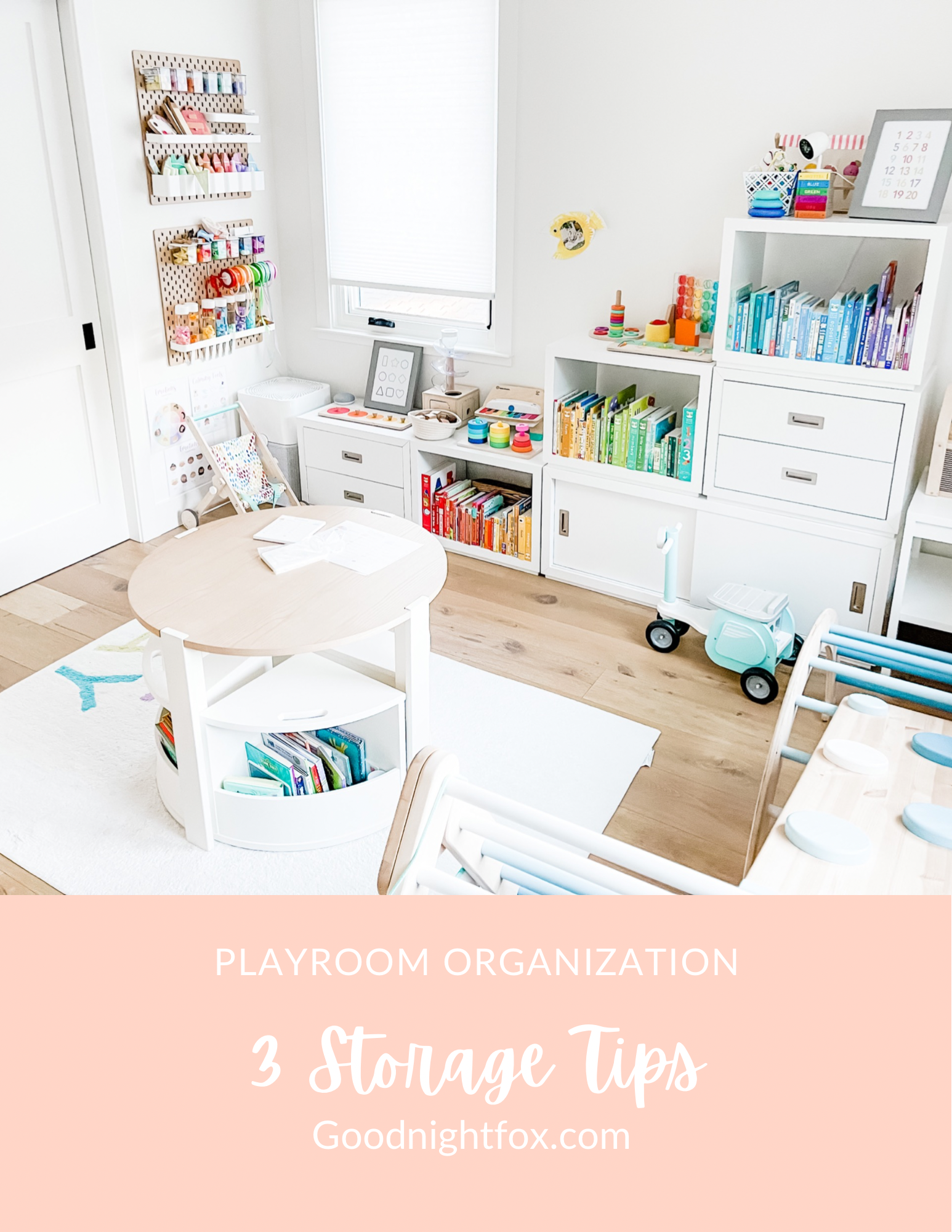The image is the cover of a blog post titled "Playroom Organization 3 Storage Tips" from goodnightbox.com. The text, which includes "Playroom Organization" in all capital letters using a sans-serif font and "3 Storage Tips" in a cursive font, is all displayed in white on a peach-colored rectangle at the bottom of the photograph. The URL is also in a sans-serif font with only the "G" in "Goodnight Box" capitalized. The background of the image is a white, modern playroom featuring dominant white color on the walls, door, window frame, and tiered shelves. The playroom has a refreshing, organized look with color-coded books arranged on white shelves, with individual sections for different colors such as blue, green, red, and orange. Some shelves are open-faced displaying neatly arranged books, while others are closed with doors and drawers. There are bulletin boards with hanging baskets full of items on the wall by the door, and a hardwood floor adds warmth to the predominantly white space. A small, round, white table sits on a white carpet on the floor, complementing the overall clean and modern aesthetic.